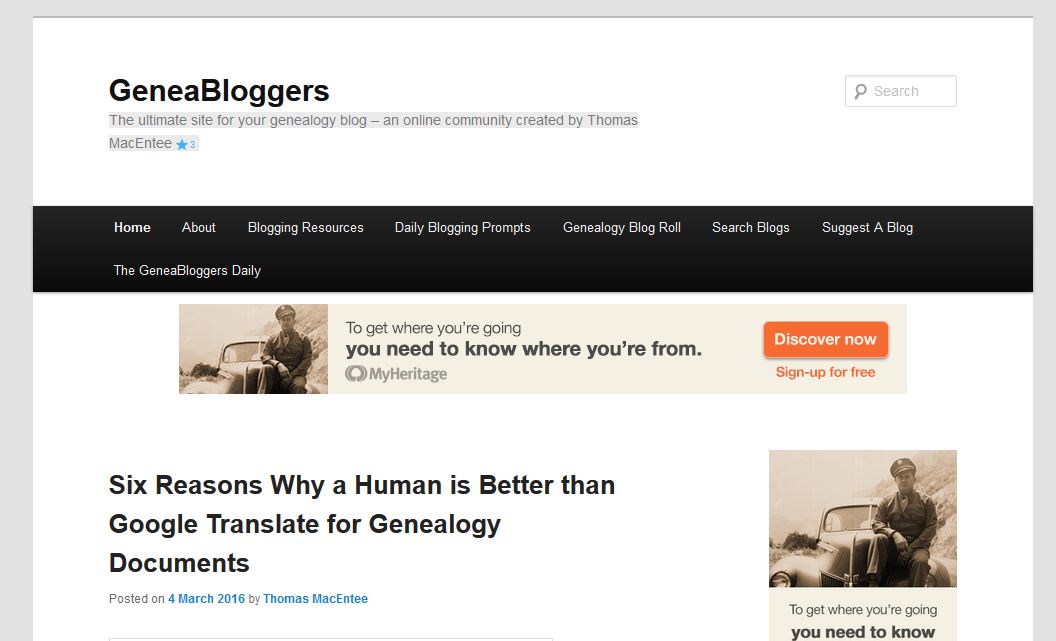This is a detailed description of the website screenshot:

The screenshot captures the homepage of a website with a gray border on the right, left, and top. Within this border, the upper section features a white rectangular banner with bold black text that reads, "Genie Bloggers: The Ultimate Site for Your Genealogy Blog – An Online Community Created by Thomas McEntree." Adjacent to the right of this banner is a smaller rectangular search field. The search field includes a gray magnifying glass icon and the word "Search" in gray font.

Directly below this, there's a navigation bar with a black background. The navigation bar contains clickable options in white text: Home, About, Blogging Resource, Daily Blogging Prompts, Genealogy, Blog Roll, Search Blogs, Suggest a Blog, and The Genie Blogger Daily.

Positioned underneath the navigation bar is a banner advertisement with a beige background. On the right side of the ad, there is a black-and-white photograph of a man in a military uniform sitting on the hood of a jalopy. To the right of this image, the text reads, "To get where you're going, you need to know where you're from." Below this slogan, "My Heritage" is displayed. Further to the right of this, a red bar presents the call-to-action text, "Discover Now. Sign up for free."